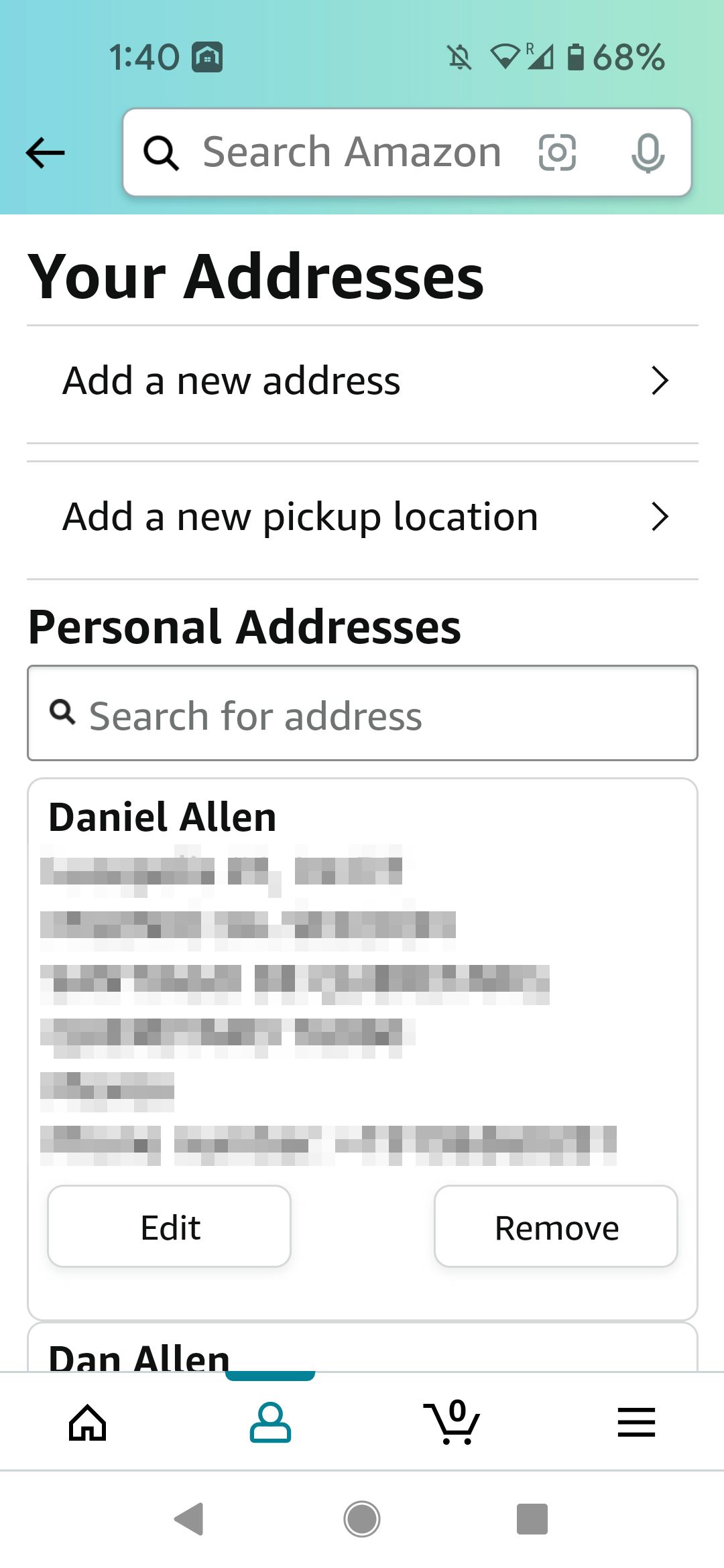This screenshot, captured from the mobile version of Amazon, prominently features the "Your Addresses" section of the website. At the top, a teal, light aquamarine-colored header houses a search bar. Positioned above the search bar are a 68% battery icon on the top right and a time stamp displaying 1:40 PM on the top left.

The main content displays two functional lines below the "Your Addresses" header: "Add a new address" and "Add a new pickup location." The second section, "Personal Addresses," includes a field for typing in a new address.

Below this address entry bar, there's a small box displaying the name "Daniel Allen" at the top, with most of the box's content redacted for privacy. At the bottom of this box, two buttons are situated: an edit button on the left and a remove button on the right.

Finally, a footer runs along the bottom of the screen, featuring several icons. From left to right, these include a house icon, a profile silhouette highlighted in green, a shopping cart icon displaying '0', and three horizontal lines indicating a menu on the far right.